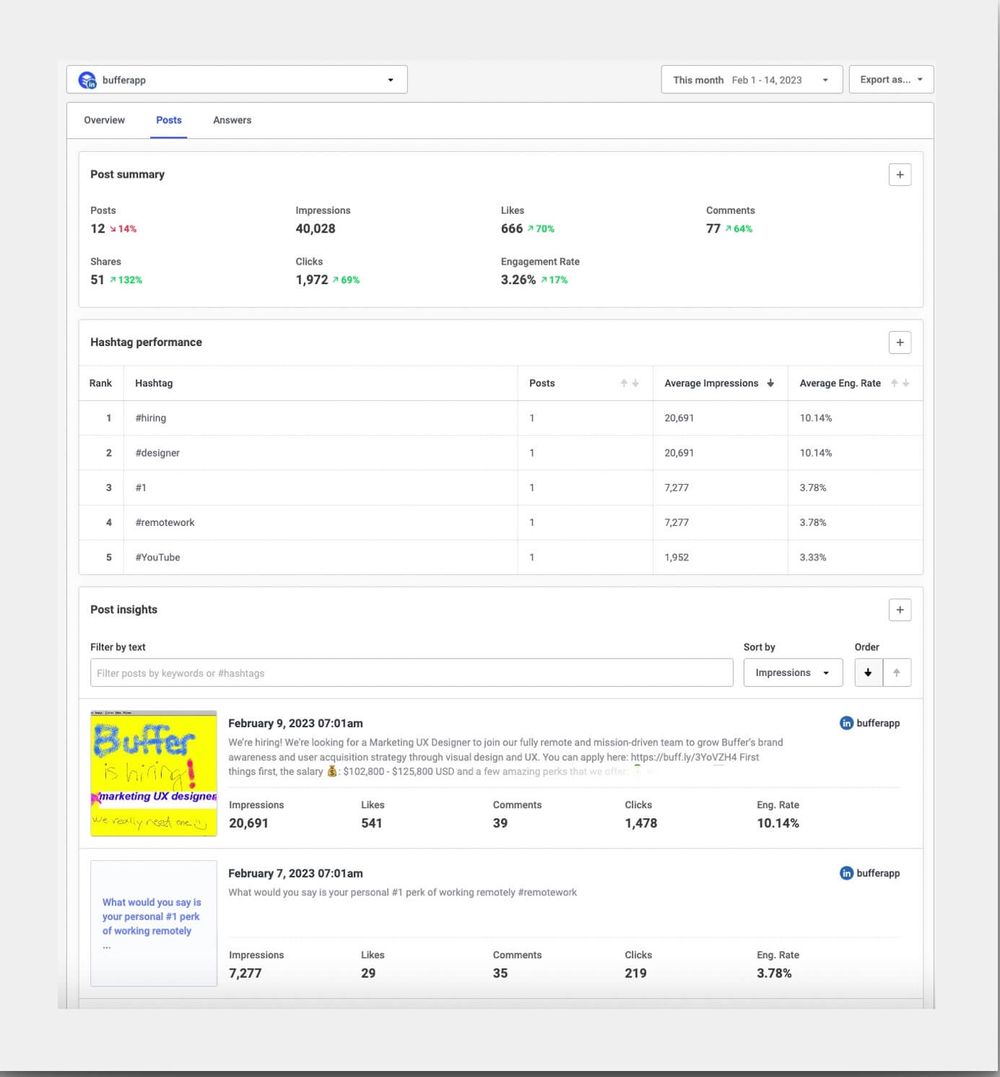This image is a screenshot taken from a computer screen with a light gray background and a predominantly white central area. At the top of the screen, there is a search bar or drop-down menu labeled "Buffer App," accompanied by an icon. Below this, there are distinct sections labeled "Overview," "Posts," and "Answers."

The "Posts" section includes summaries with black areas featuring various numbers. There are also colored indicators, with some areas in red and others in green, indicating different statuses or metrics.

Further down, there is a section titled "Hashtag Performance," which resembles a spreadsheet. This section lists columns such as "Rank," "Hashtag," "Posts," "Average Impressions," and "Average Engagement Rates."

Scrolling down the page, there is a "Post Insights" section, highlighted by a yellow box containing the message "Buffer is hiring." At the very bottom, there is another box with the question, "What would you say is your personal number one perk of working remotely?"